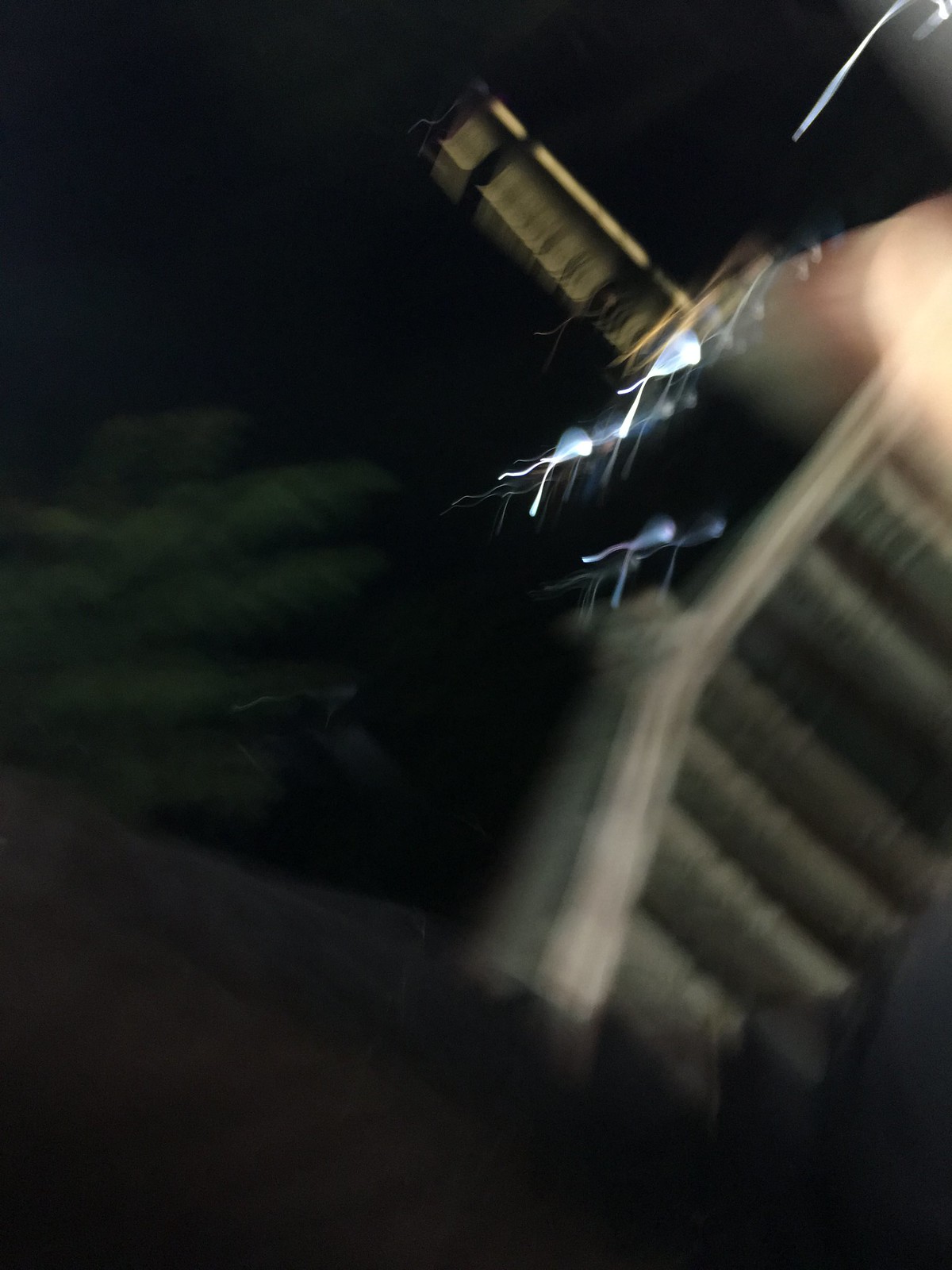A blurry photograph with a predominantly black background, features a complex and somewhat ambiguous scene. Amid the dark backdrop, there are elements in copper and black, creating a slightly metallic appearance. A flesh-toned object is visible, standing out against the darker hues. Scattered throughout the image are small, white, elongated figures resembling tiny swimming fish, or even miniature octopuses with many legs. On the left side of the frame, a tree-like shape is discernible, providing a stark contrast to the surrounding elements. A brown structure, which has a prominent top and column-like extensions, appears both in the foreground and partially overlays some aspects of the scene. This mixture of elements gives the impression of an underwater environment, possibly a fish tank, with various decorative and organic components melding together in the limited clarity of the image.